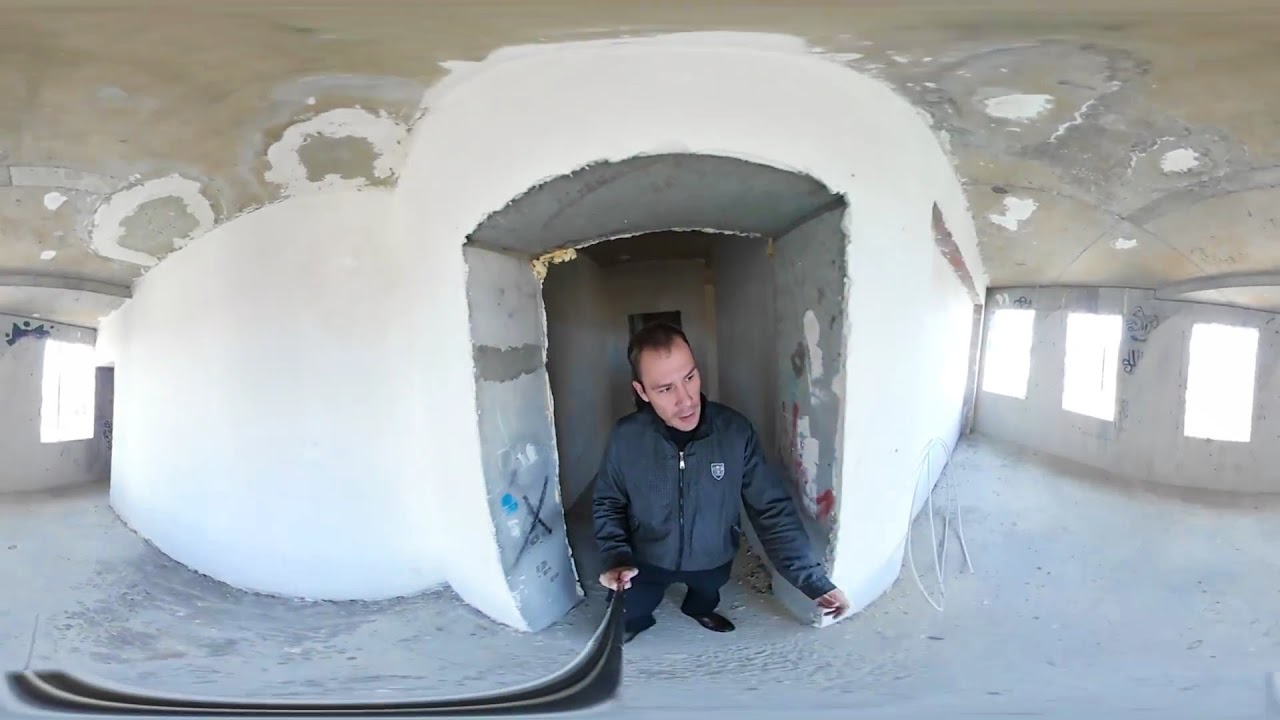This image captures a scene of a man standing at the entrance of what appears to be an unfinished or abandoned building, suggesting a place either under construction or in desperate need of restoration. The structure is predominantly white, featuring unpainted drywall on the walls. The ceiling is a tan-brown color adorned with patches and spots of white paint, and it has circular outlines that might be for future lighting installations. 

The man, central to the image, is in the doorway of what looks like an igloo-shaped structure within the larger building. He wears a light gray jacket with a small logo on it, dark blue pants, and black dress shoes. His jacket is zipped up in the front. 

On the right side of the room, there are three windows, and a fourth window is partially visible behind the igloo-like structure. The walls show signs of neglect or preparation for further work, with scattered spots of paint and an 'X' marking in black. A symbol or wording is noted between or next to the windows, adding to the unfinished aesthetic of the space. The floor is white and likely tiled, complementing the overall stark, incomplete look of the environment, indicating that the building has been abandoned or needs significant renovation.